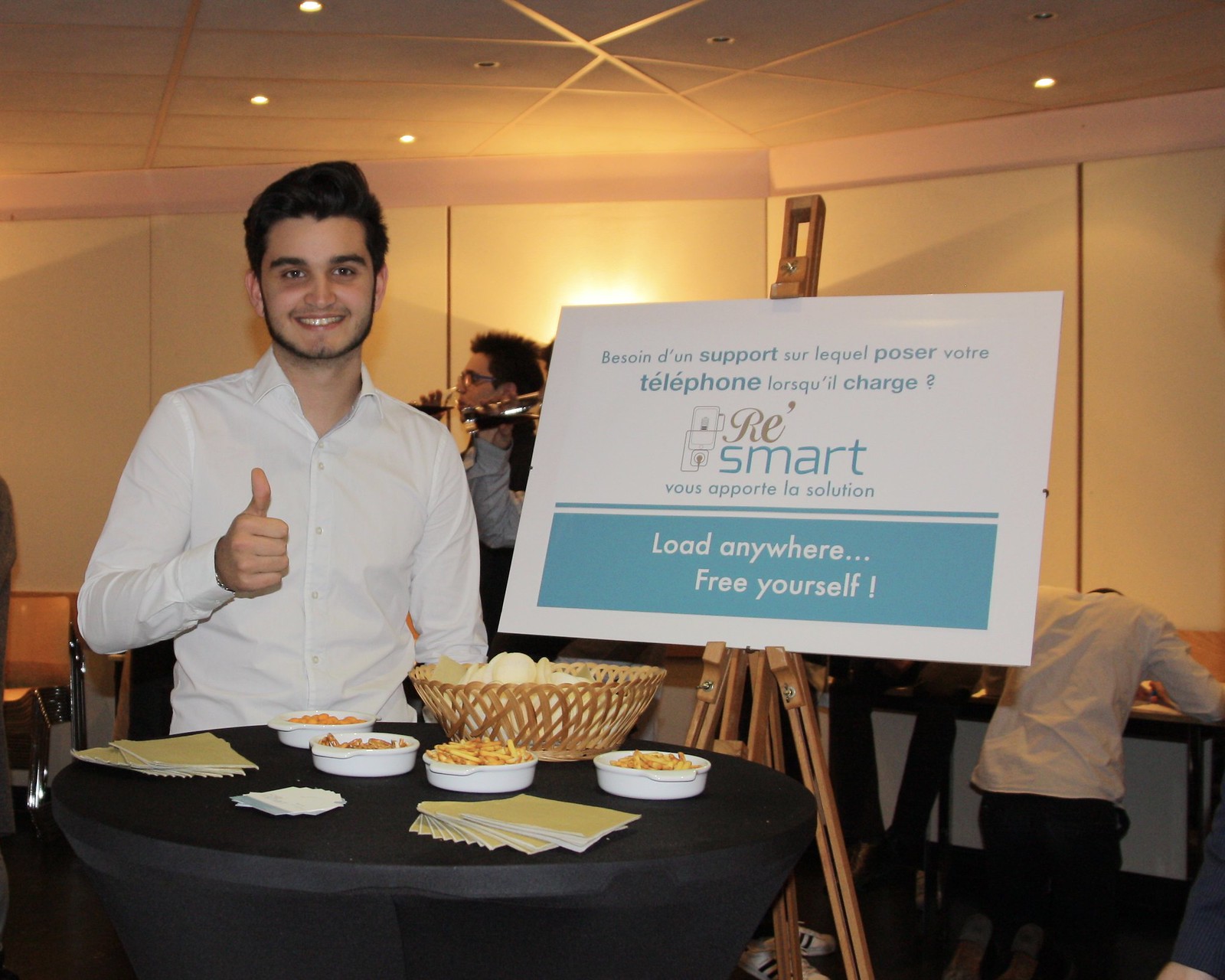At what appears to be a lively conference or event, a young, tan-skinned man with facial hair and silky, curly dark hair stands behind a round table draped with a black tablecloth. His white button-down dress shirt accentuates his welcoming smile as he gives a thumbs-up sign. The table is adorned with an assortment of snacks, including a large basket of chips and several smaller bowls filled with bar-style nibbles, along with various napkins.

The ambiance suggests a lounge or a bar-like setting, with several attendees visible in the background. Some are bent over another table, seemingly writing, eating, or perhaps engaged in conversation. The majority appear to be men. A prominent placard next to the man showcases text primarily in French, though it also features English phrases like “Load Anywhere, Free Yourself” and “You’re as opportune to solution.” The colors prominently featured in the scene include black, white, gray, yellow, orange, pink, and blue, adding to the vibrant atmosphere of the event.